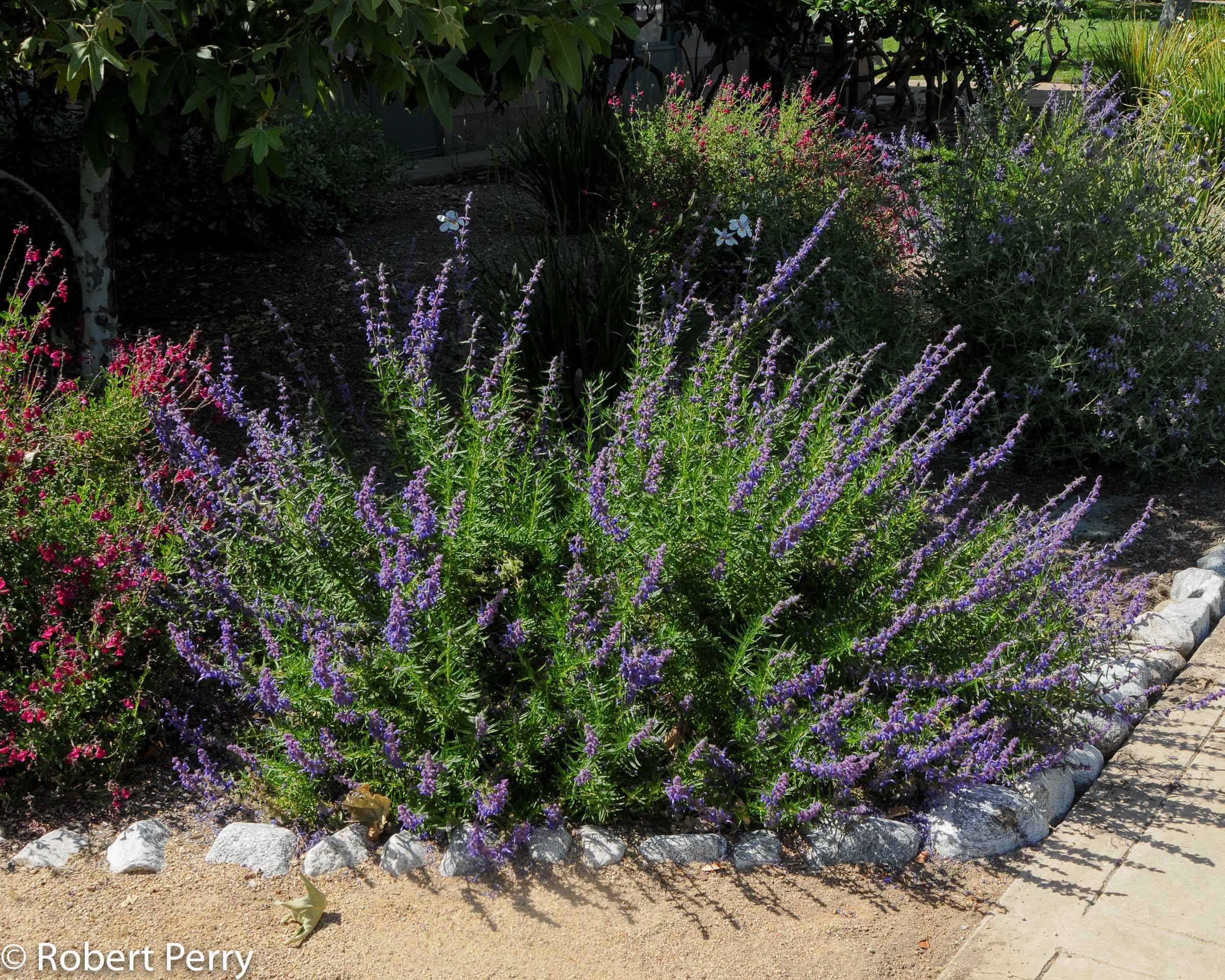In this vibrant daytime garden photograph taken by Robert Perry, a neatly organized bed of multicolored bushes is prominently featured. The scene is framed by a stone border in shades of off-white and tan, creating a clear division between the lush greenery and the clean pavement to the right. The bushes display a rich array of colors, including light violet and pink flowers set against dark and light green foliage. The garden area also includes patches of sand and soil, and is set against a backdrop of towering trees, adding depth to the composition. The text "Robert Perry" is discreetly placed in white at the bottom left of the image, identifying the photographer. Overall, the image captures a meticulously arranged garden scene viewed from a straight-on perspective, emphasizing the natural beauty and attention to detail in the landscaping.